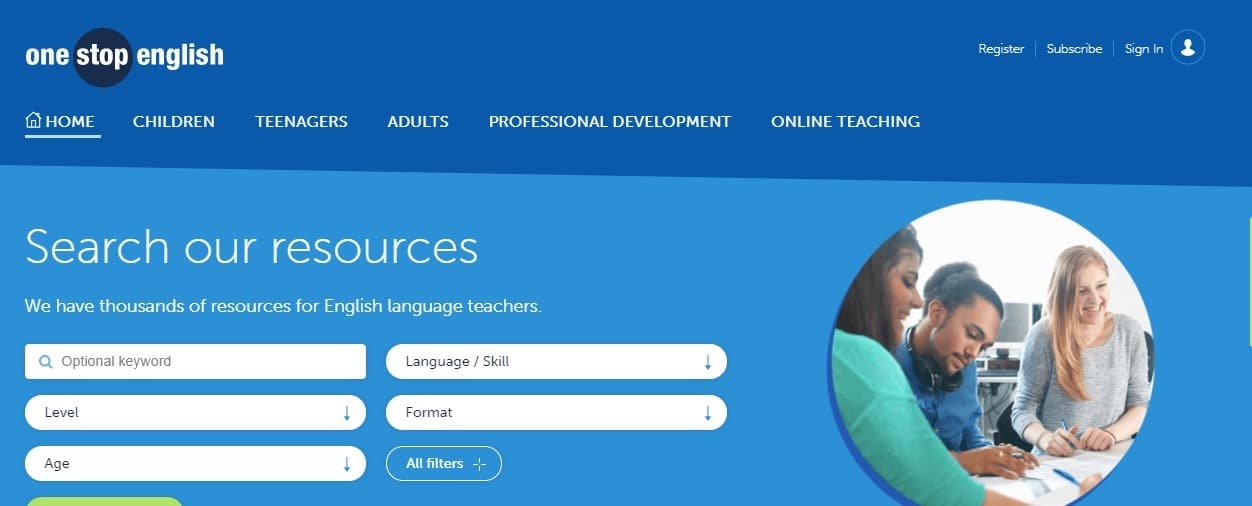This is a detailed screenshot from the "One Stop English" website. The page features a navy blue top header with the "One Stop English" logo located in the top-left corner, where the word "stop" is highlighted with a black circle. In the top-right corner, there are links for "Register," "Subscribe," and "Sign in," formatted as plain text.

Below the header is a menu bar with the following options listed from left to right: "Home," "Children," "Teenagers," "Adults," "Professional Development," and "Online Training." This menu is situated against a blue background.

Underneath, to the left side of the screen, the text "Search our resources" is presented in white. Directly below this text, there's a search bar for keyword entry, accompanied by filter bubbles for criteria such as "Level," "Age," "Language," "Skill," and "Format," each with a downward arrow for additional selection options. An "All Filters" tag is also visible in this section.

On the right side of the screenshot, there's an image depicting a classroom setting. In this photo, a man is centrally positioned and appears to be writing something on a desk. The image serves as a visual complement to the educational theme of the website.